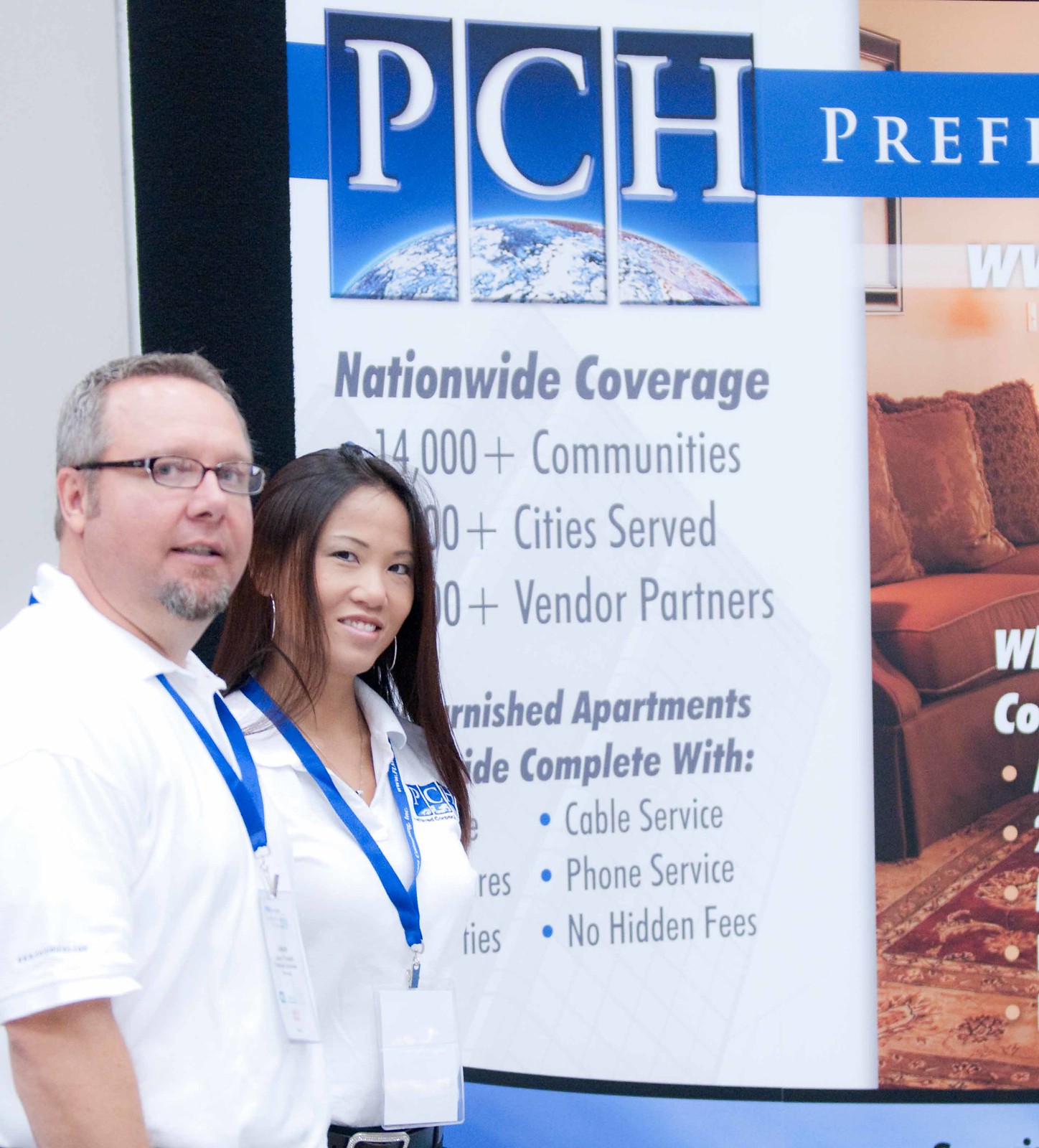The rectangular photograph features a man and a woman, both dressed in white polo shirts bearing blue lanyards and ID badges. Positioned in front of a partially visible poster, the shirts and the sign both sport the PCH logo, which includes the letters P, C, and H inside individual rectangles, with "Preferred" suggested below. The backdrop advertises services for nationwide coverage, listing 14,000+ communities, numerous cities served, many vendor partners, and furnished apartments with comprehensive amenities such as cable, phone service, and no hidden fees. The man, slightly taller with short salt-and-pepper hair, glasses, and a goatee, stands beside a slightly shorter Asian woman with shoulder-length dark hair and silver hoop earrings. To the right of the poster, a living room scene features the edge of a couch and a Persian rug, adding context to the services being promoted.